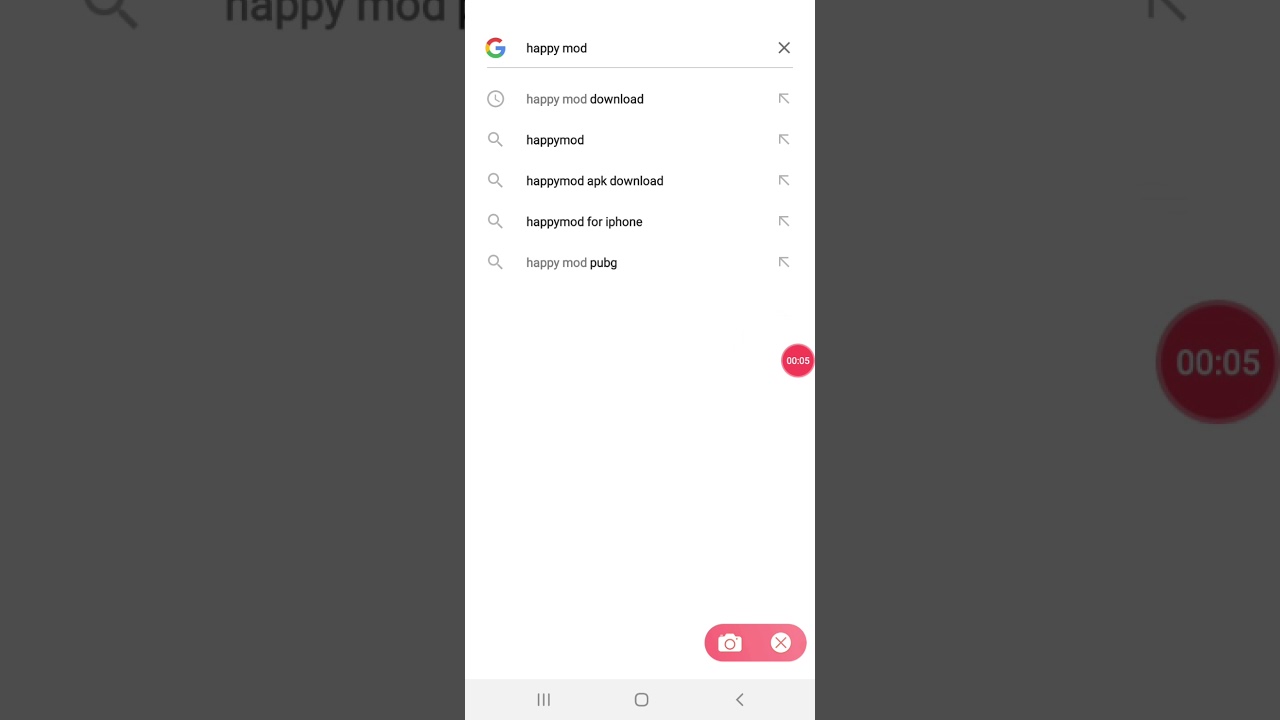In the screenshot image, there are three distinct columns. The farthest column to the left is a gray rectangle that contains partially visible text at its top, likely "happy" and "mod" (M-O-D), though the text is cut off due to the image's cropping.

The middle column prominently features the Google logo followed by the search query "happy mod" in lowercase black text. 

On the right side of this column is a cancel button. 

Below the central search bar are several search suggestions, each preceded by a magnifying glass icon. These suggestions include:
- "happy mod download"
- "search for happy mod"
- "happy mod APK download"
- "happy mod for iPhone"
- "happymod plugin"
  
To the right of each search suggestion, there is a gray arrow icon that points to the 11 o'clock position.